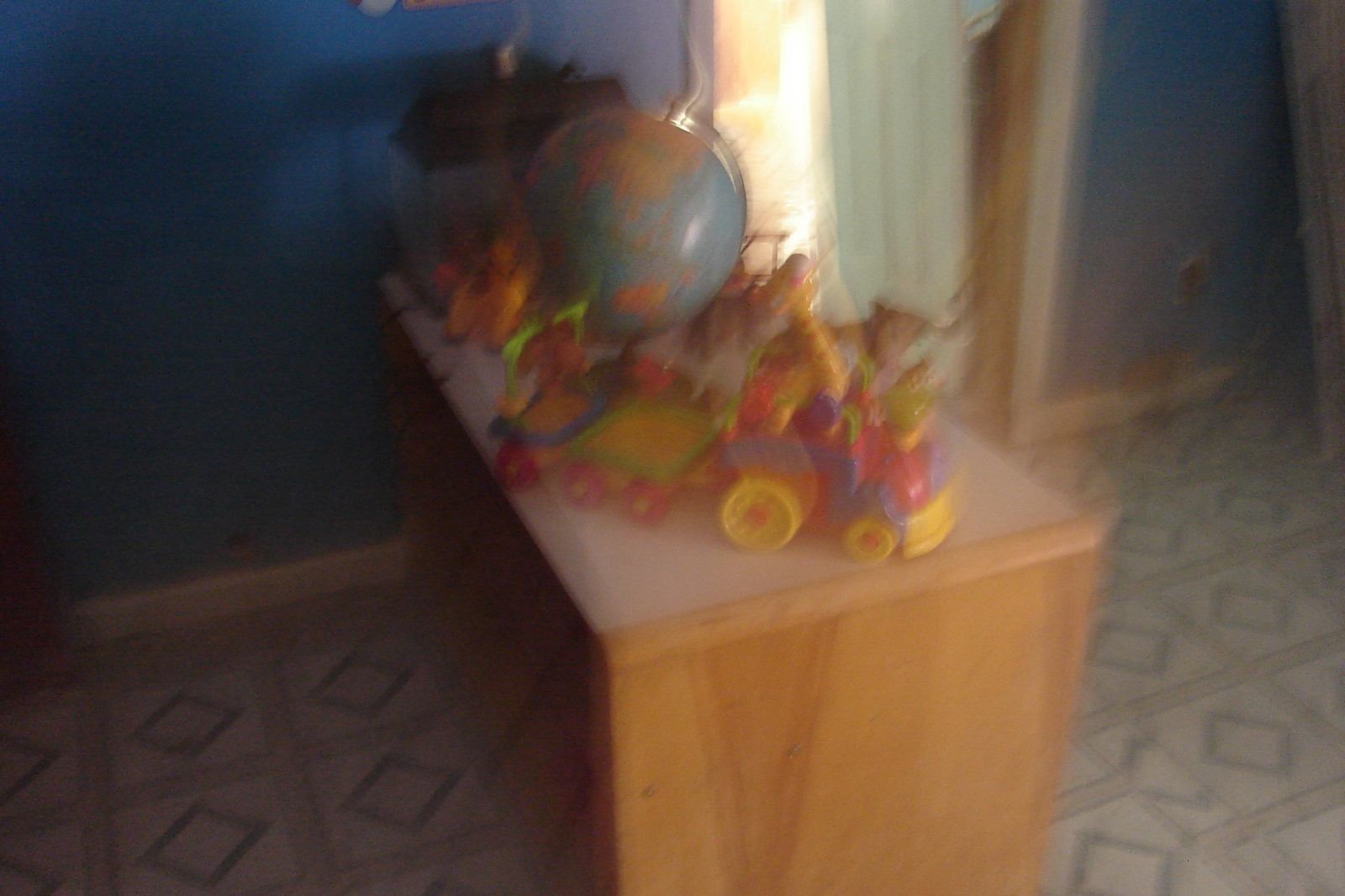In a room adorned with a blue wall that has a white edge, a wooden desk stands prominently beside an open, white doorway. The floor is tiled with a pattern of white squares accented by blue and red detailing. On the desk, a collection of colorful children's toys is displayed, featuring items with yellow wheels and hues of pink, purple, red, and blue. Among the toys, a globe is prominently visible, illustrating blue oceans and continents colored in yellow, orange, and other shades. The desk also seems to hold a multicolored train filled with toy animals. A window in the middle of the wall, dressed with a partially open white drape, allows light to stream in, casting a gentle glow across the scene. Despite the slightly blurry photograph, the playful setting and its vibrant elements are unmistakable.